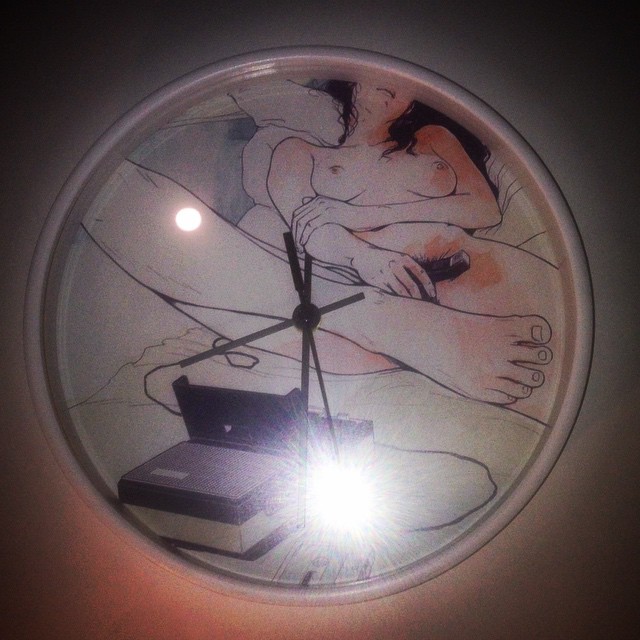This image features a round analog clock with sleek black hour, minute, and second hands. Notably, the clock face lacks numerical markings. Behind the clock, there is an intriguing vintage cassette recorder, characterized by its slim buttons for functions such as stop, pause, and eject. The cassette compartment is open, revealing the interior mechanics. 

Dominating the backdrop is an artistic photograph of a nude woman with long black hair. She is poised gracefully on what appears to be a white bedspread, her right leg curled up to touch her left leg, while her left hand rests on her right elbow. Her breasts are visible, and she holds a microphone connected to the recorder in her right hand, positioned just above her pubic region. The meld of technology with the intimate and raw human form creates a striking and evocative composition.